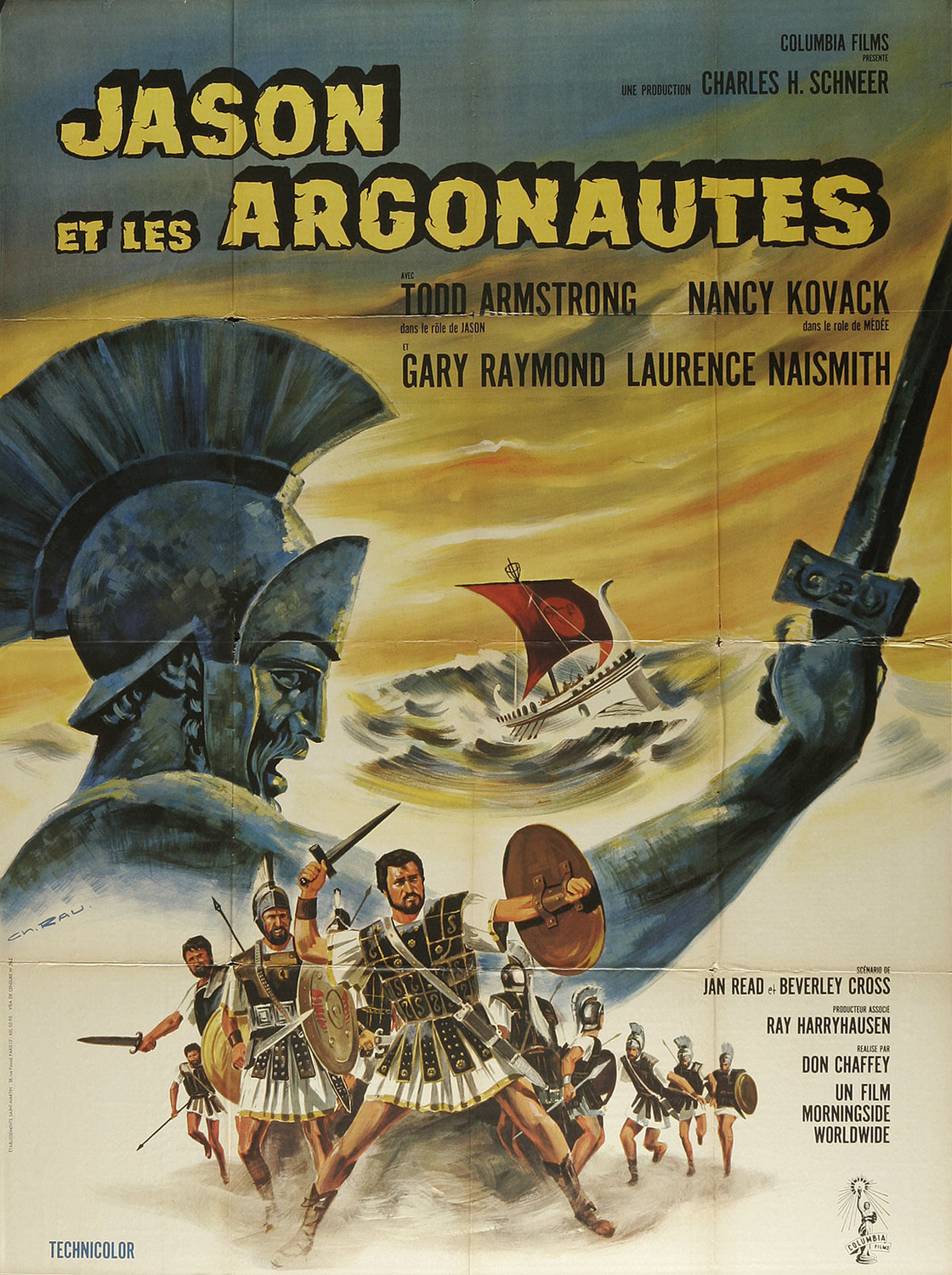The movie poster, titled "Jason Et Les Argonautes" in bold yellow letters at the top, features prominent actors' names in black text, including Todd Armstrong, Nancy Kovack, Gary Raymond, and Lawrence Naismith. The sky forms a blue and yellow backdrop, highlighted by the Columbia Films logo and mentions of Charles H. Schneer. Dominating the poster is an artistic depiction of a white Viking boat with a red sail navigating choppy waters, rendered in striking hues of white, yellow, and blue reminiscent of oil painting.

To the left, a dark-colored statue of a Roman gladiator poised in profile commands attention. The statue, draped in classic gladiatorial gear, wields a metal sword with an outstretched arm. At the bottom of the poster, a group of gladiators, dressed in white robes with brown leather boots, brandish shields and swords, ready for battle. Additional text near the bottom left corner notes "Technicolor," and the names Ian Reed, Beverly Cross, Ray Harryhausen, Don Chaffey, and Morningside Worldwide are listed in black. A small Columbia Pictures logo completes the composition at the bottom right, cementing its cinematic grandeur.